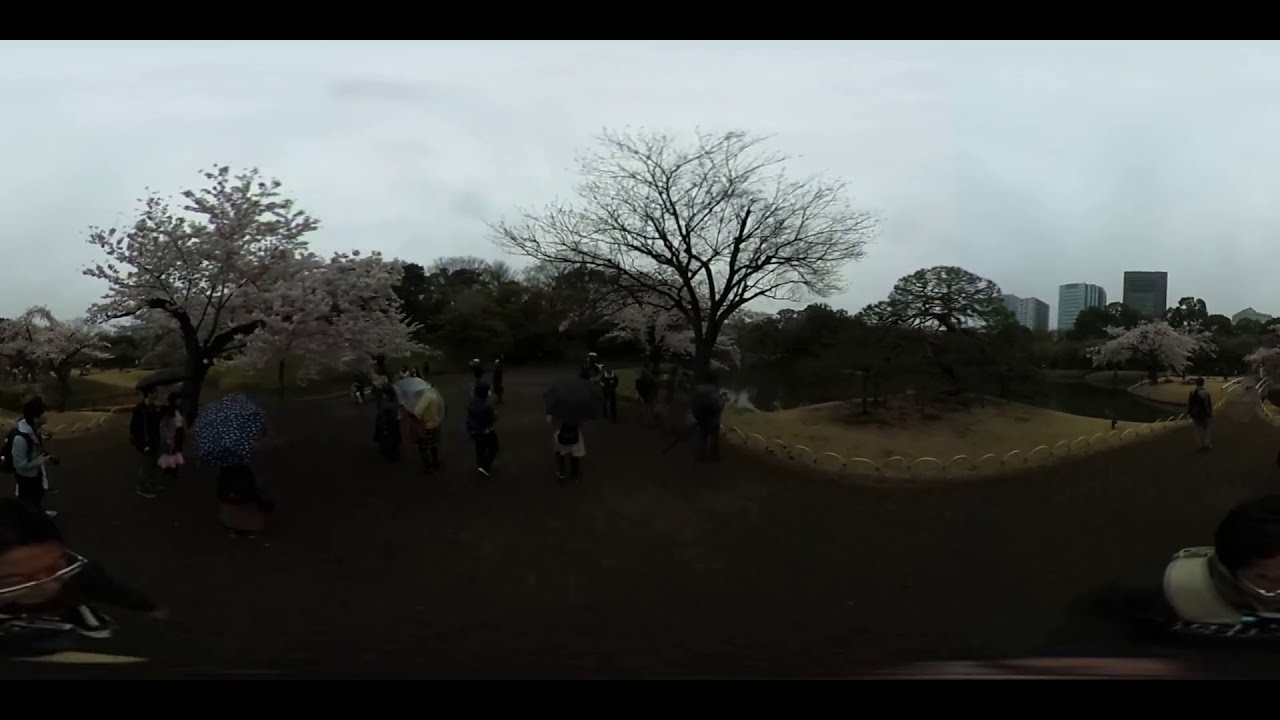The horizontal rectangular photograph, bordered by thick black stripes at the top and bottom, depicts a dimly lit, overcast scene in a park. The sky is mostly a blend of gray and white, casting a gloomy ambiance over the setting. In the middle distance, approximately 20 people, dressed in long sleeves and pants, gather. Some carry umbrellas, suggesting possible rain. They stand on a paved walkway that is bordered by grass and various trees. To the right center, there is a sandpit surrounded by a short stone wall and adorned with a few trees, one of which has pinkish leaves, possibly a cherry blossom. Most other trees are bare, indicating a fall or early winter timeframe. In the background, to the upper right, several buildings hint at a nearby city, providing a stark contrast to the natural surroundings of the park. The overall scene is muted in tones of gray, black, beige, and white, emphasizing the late afternoon light and cloudy sky.